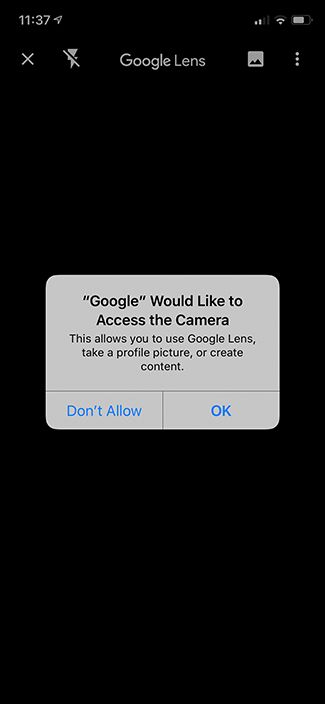A mobile phone screenshot predominantly features a solid black screen with minimal activity displayed. At the very top of the screen, the time is shown as 11:37 AM. The status indicators on the top-right reveal two bars for cellular connectivity, two bars for Wi-Fi signal strength, and approximately 75% battery life remaining. The user is currently within the Google Lens app, as denoted by the app’s name centered at the top. Accompanying the app's name are several icons: a picture clipart and three vertical dots for a menu on the right, a flash icon with a slash indicating the flash is off to the left, and a small 'X' icon to exit the feature further to the left.

A prominent light gray popup with rounded corners is centered on the black screen, overlaying the background. The popup reads, "Google" would like to access the camera," in quoted text. Below this, a smaller font explains, "This allows you to use Google Lens, take a profile picture, or create content." At the bottom of the popup are two options for the user: a blue "Don't Allow" button on the left and a bolder "OK" button on the right.